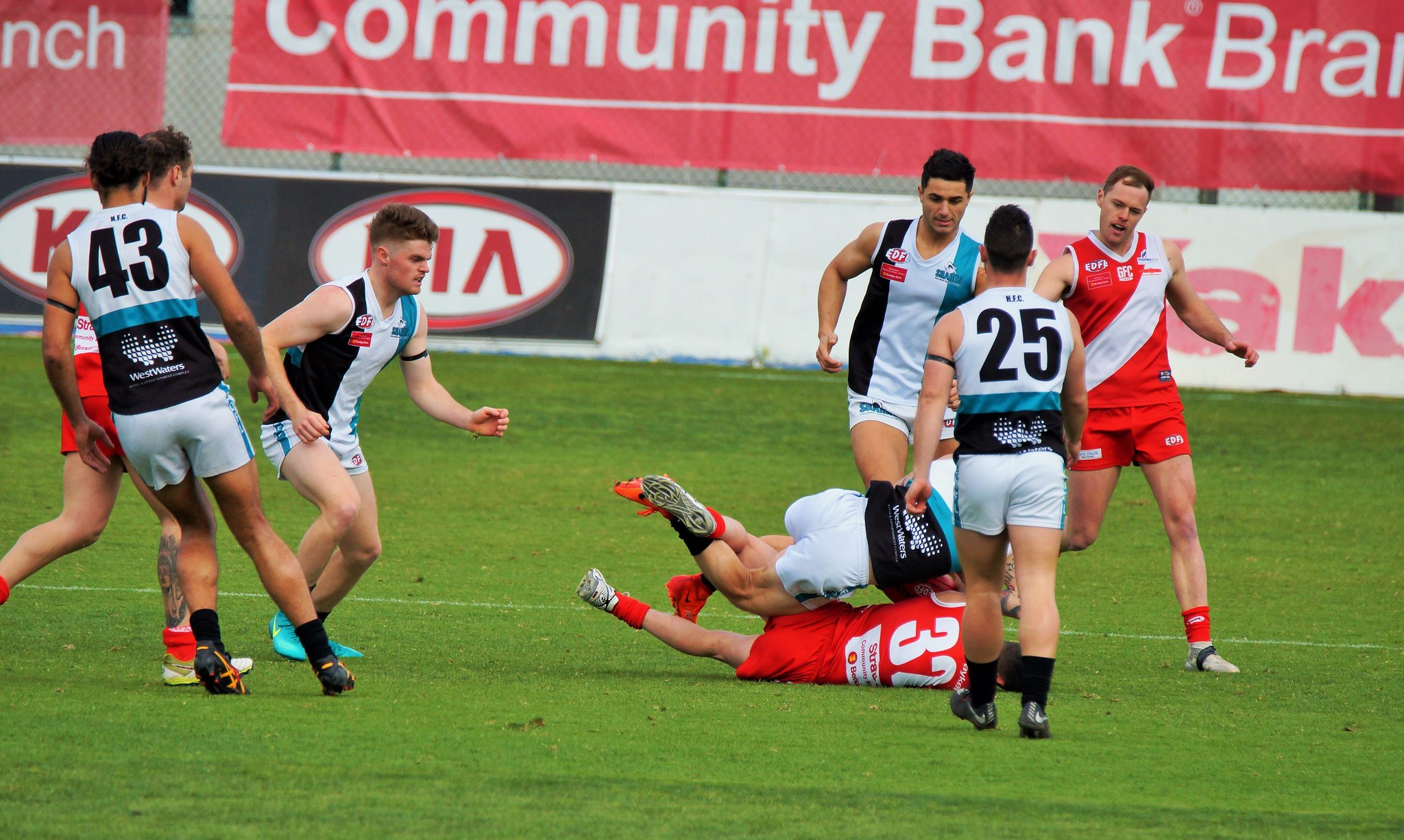In this detailed, horizontal photograph of an outdoor rugby match, set on a vivid green grass field during daylight, we observe eight male players dressed in distinct uniforms. On the left side of the image, three players are visible: two are wearing black, white, and blue uniforms, while one is in a red and white uniform. The player in the black, white, and blue uniform closest to the viewer is identified by the number 43 on his back. On the right side, the composition continues with five more players: three donned in black, white, and blue uniforms and two in red and white uniforms. Number 25, a player in a black, white, and blue uniform, is also seen facing away from the viewer.

A dynamic scene unfolds as number 32, a player in a red and white uniform, lies on the ground with another player in a black, white, and blue uniform atop him, although this latter player's number remains unseen. The other players appear to be running and directing their attention towards the two on the ground. 

In the distance, a white wall adorned with advertisements occupies the background, prominently featuring the Kia logo and a largely legible red banner reading "Community Bank Branch." Another partially obscured advertisement with the letters A and K is also visible. This image captures an intense moment in the match, highlighting the competitive spirit of the players against the backdrop of vivid colors and visible branding.